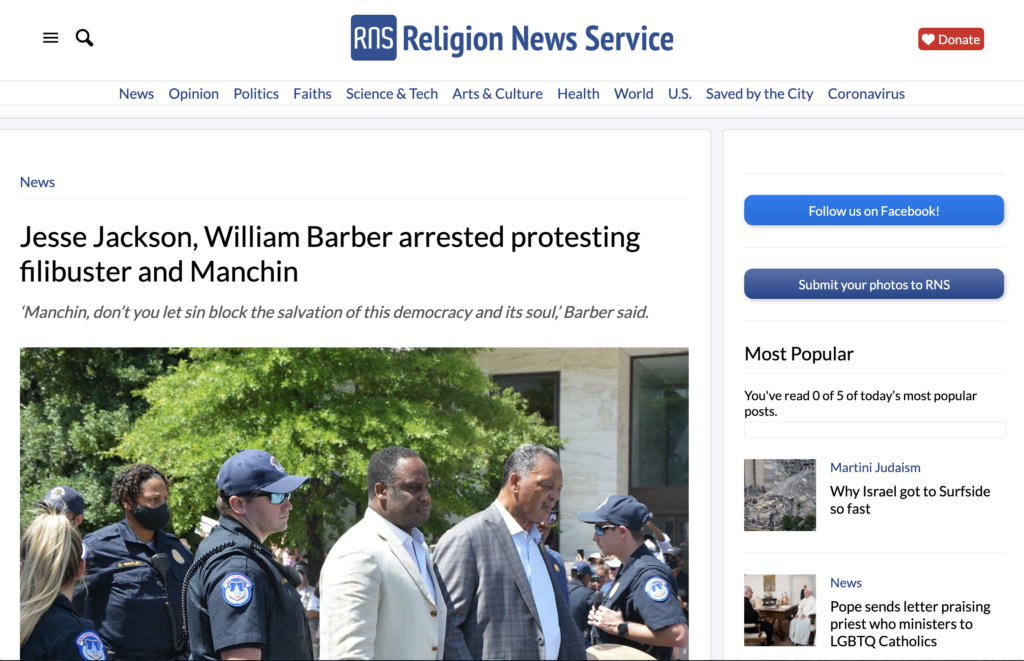A detailed caption for the provided image could be:

"The image depicts a web page from the Religion News Service (RNS). In the upper left corner, there is a menu icon represented by three horizontal lines next to a magnifying glass icon for the search bar. Adjacent to these, a blue square logo with 'RNS' in white lettering is visible, and the full name 'Religion News Service' is written in blue type next to it. To the right of the logo, a prominent red button with 'Donate' is displayed, featuring a white heart icon.

At the top of the page, there is a navigation bar with several tabs in blue text: News, Opinion, Politics, Faiths, Science and Tech, Art and Culture, Health, World, US, Saved by the City, and Coronavirus. Just below the navigation bar, a blue button invites users to 'Follow Us on Facebook.' Another button, dark blue, encourages visitors to 'Submit Your Photos to RNS.'

Dominating the central portion of the web page is a headline reading 'Jesse Jackson, William Barber arrested protesting filibuster and Manchin,' followed by a quote attributed to Barber: 'Manchin, don’t you let sin block the salvation of this democracy and its soul.' Below this headline, a 'Most Popular' section lists popular articles, and a photograph shows Jesse Jackson and William Barber being detained by authorities during their protest."